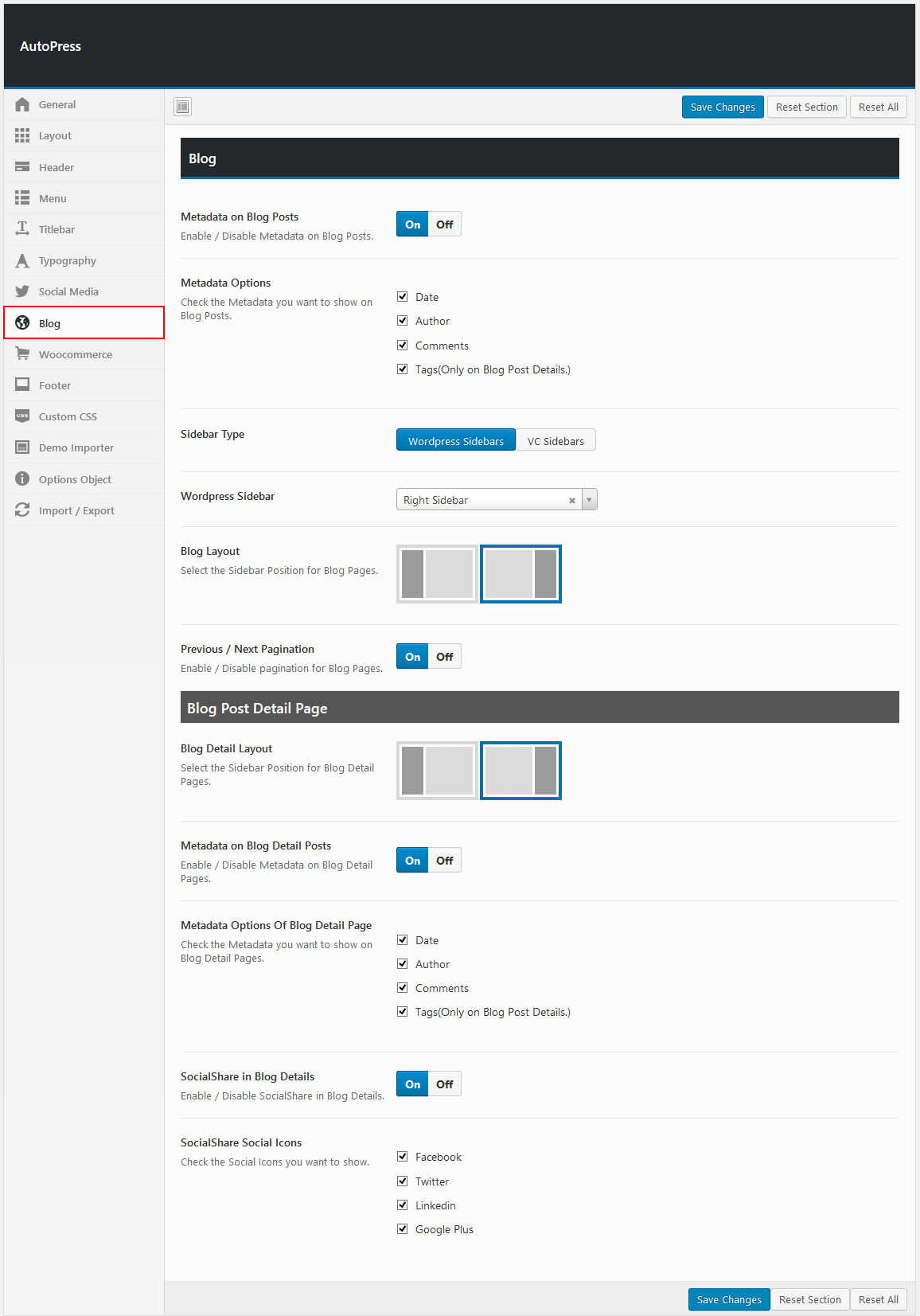This screenshot captures the "Settings" or "Changes" section of the Autopress website. The interface is framed by a black border along the top left, which prominently displays the word "Autopress." Below this, a gray sidebar provides a navigation panel starting with "General" and followed by: "Layout," "Header," "Menu," "Sidebar," "Typography," "Social Media," "Blog" (the current section), "Footer," "Custom CSS," "Demo Importer," "Options Object," and "Import/Export."

On the right side, the interface features several control options including "Save Changes," "Reset Section," and "Reset All." 

Within the "Blog" section, various settings are configured:
- **Metadata on Blog Post**: Toggle option set to "On"
- **Metadata Options**: Checkboxes for "Date," "Author," "Comments," and "Tags Only" are all selected.
- **Sidebar Type**: Options for "WordPress Sidebar" and "VC Sidebar," with "WordPress Sidebar" chosen.
- **Sidebar Position**: Dropdown menu set to "Right Sidebar."
- **Blog Layout**: Configured to display the sidebar on the right side.
- **Pagination**: Toggle for "Previous/Next pagination" is turned on.
- **Blog Post Detail Page**: Layout settings for Blog Detail Pages with the sidebar on the right.
- **Metadata Detail Post**: Toggle switch is on.
- **Metadata Options of Blog Detail Page**: Checkboxes labeled "Date," "Author," "Comments," "Tags Only," are all selected.
- **Social Share and Blog Details**: Toggle set to "On"
- **Social Icons**: Checkboxes for "Facebook," "Twitter," "LinkedIn," and "Google+" are all selected.

At the bottom of this section, controls for "Save Changes," "Reset Section," or "Reset All" are available for finalizing or discarding changes.